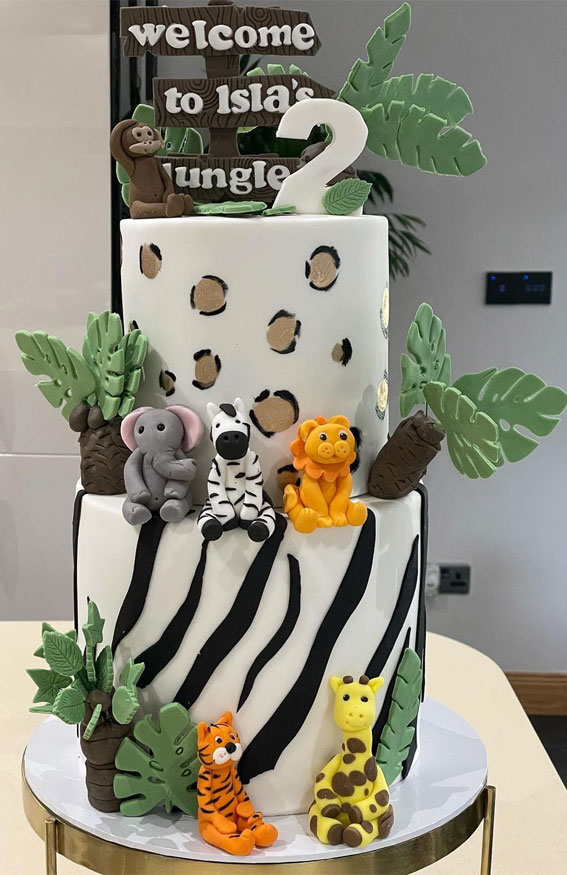This image depicts a very large, multi-tiered birthday cake sitting on a cream-colored table with a white top and a gold metallic base. The cake itself is white and has two cylindrical tiers. The bottom tier is much larger, decorated with black zebra stripes, and features a figurine of a sitting tiger and giraffe at its base. There are also green palm trees on either side of the cake.

The upper tier of the cake is slightly smaller and shorter, adorned with black and tan spots scattered across its surface. Sitting on the edge of this tier are figurines of an elephant, zebra, and lion, all in a seated position. On top of this tier is a wooden signboard with a welcome message that reads "Welcome to Isla's Jungle," with "Welcome" on the top, "to Isla's" in the middle, and "Jungle" at the bottom. Next to the signboard, there's a white number "2" and a monkey figurine. The background features a whitewashed wall, adding a neutral backdrop to highlight the detailed and vibrant elements of the cake.